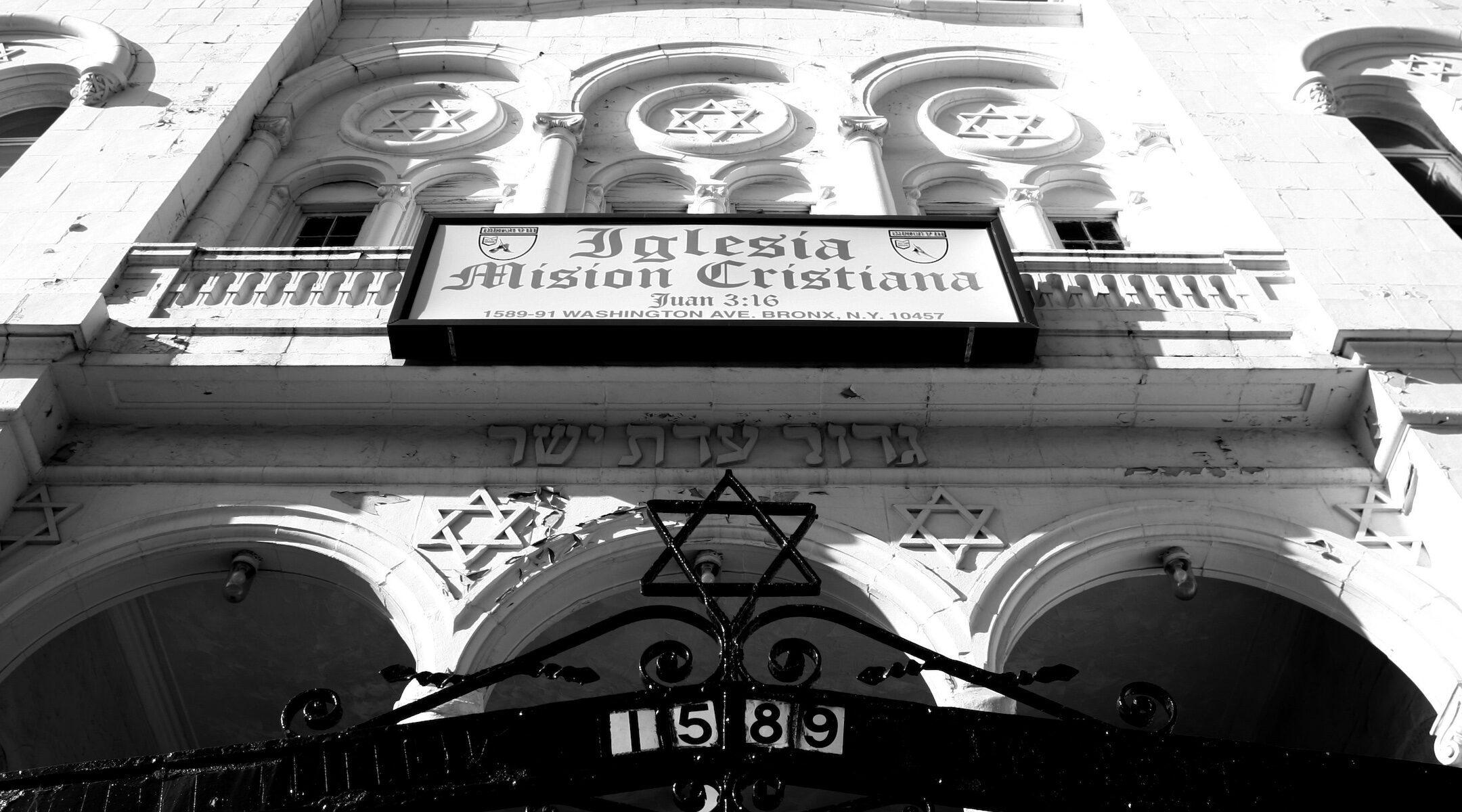This high-contrast, black and white photo features a detailed view of a white building highlighted with numerous Star of David symbols. Predominantly visible is a sign framed in black, reading "Iglesia Misión Cristiana 1316" along with the address "1589-91 Washington Avenue, Bronx, NY 10457." Positioned centrally on the building, the sign sits above three arches, each crowned with a Star of David enclosed in a circle. Flanking these arches are additional windows, each adorned with another Star of David. Below the sign, Hebrew writing is seen amidst multiple Star of David symbols, some partially obscured by connecting pillars. The structure appears to be made of brick, with further details including a metal gate in the foreground, intricately designed with ironwork and prominently displaying the number "1589." The vantage point of the photograph is upward, adding to the grandeur and intricacy of the building's facade.